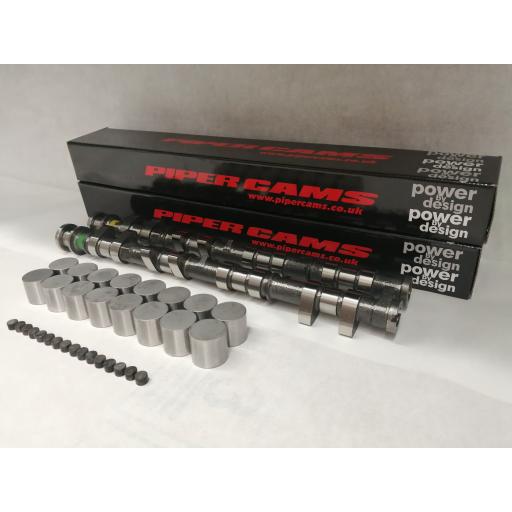The image displays a gray backdrop and surface, showcasing a product prominently. At the rear, there are two long black boxes adorned with red text that reads "Piper Cams" alongside the website "www.pipercams.co.uk" and the repeated slogan "Power by Design." In front of these boxes are multiple cylindrical metal components, likely steel, organized in a structured layout. Specifically, there are two rows of eight larger silver cylinders, and in front of them, approximately twenty smaller black cylindrical items are aligned. The items appear to be interconnected parts, perhaps magnetic, indicative of their functional design. Additionally, smaller gray dot-like elements, resembling beads, are scattered in the bottom left, adding intricate detail to the overall setup.